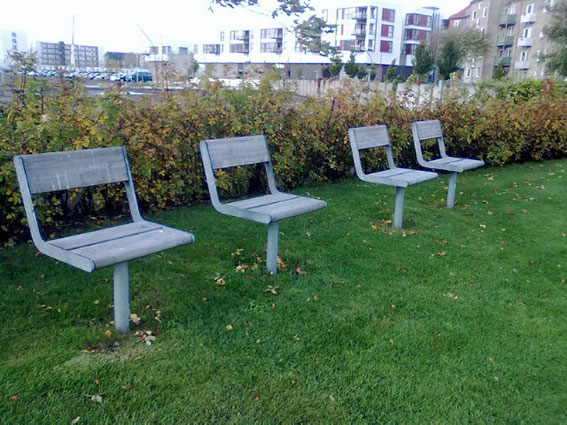In this outdoor scene, we see four identical gray chairs positioned in the grass. Each chair is attached to a gray metal pole, approximately 12 to 14 inches tall, rising from the ground. The seating structure includes two gray wooden slats for the seat and a single wooden slat for the backrest, all supported by metal frames. There is a noticeable gap between the seat and the backrest. The chairs are spaced progressively further away, viewed from an angle, rather than straight on. 

Behind the chairs, a line of bushes with yellow and green leaves serves as a natural barrier. These bushes are taller than the chairs, effectively enclosing the grassy area. In the upper right corner of the image, there is a series of tall apartment buildings, including a prominent white building with numerous windows and balconies, and a light brown building also featuring large windows and balconies. In the upper left corner, a parking lot is visible, along with additional, more distant buildings. This setup suggests the area might be a public garden or park, offering a blend of natural and urban elements.